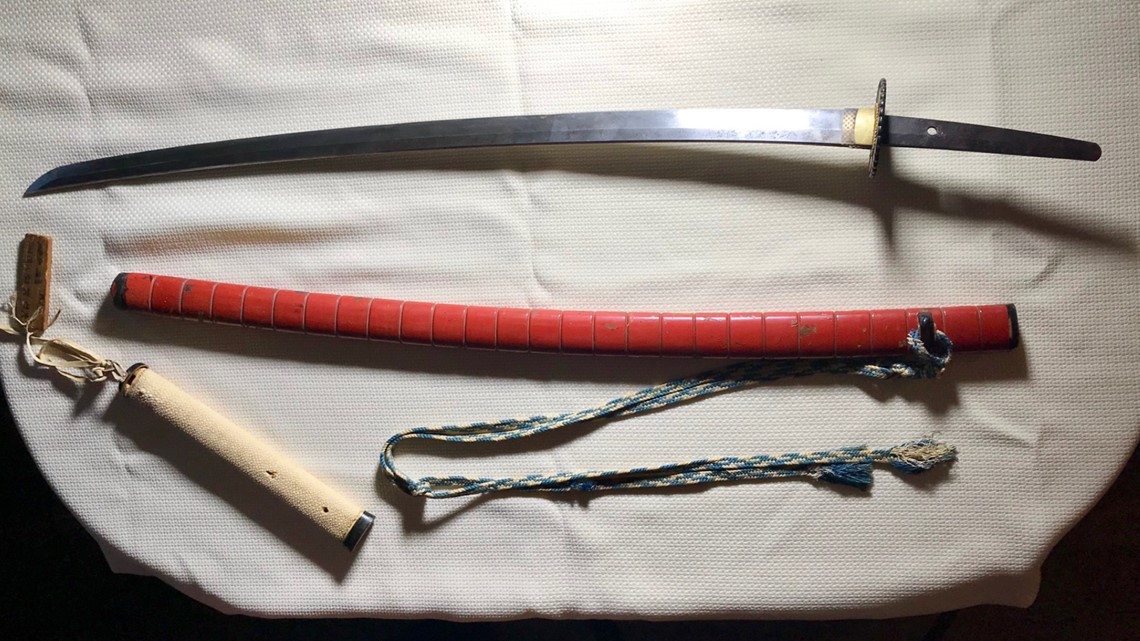In the photograph, there is a meticulously crafted black katana, partially unsheathed, its black blade and handle gleaming faintly under the low light, suggesting the image was taken at night. This striking weapon rests horizontally across a beige fabric with an intricate pattern of small squares or circles, reminiscent of a delicate vinyl tablecloth or bag. The vibrant red sheath of the katana lies beneath it, adorned with black tips and accompanied by a braided string that appears friendship bracelet-like in design, curving and frayed towards its end. Additionally, a mysterious wooden block with a red string and a white cylindrical object with a sign tied to its back can be seen, further hinting at the historical and ornamental nature of this arrangement.